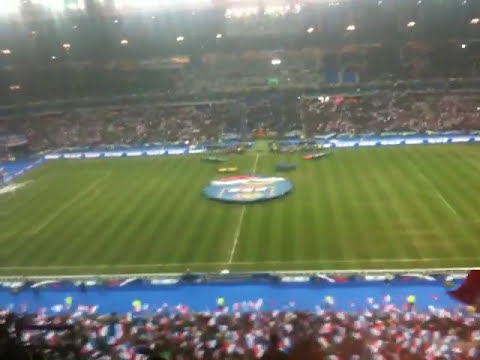This photograph depicts an outdoor stadium, likely hosting a soccer match. The massive green field at the center of the image is flanked by blue sidelines, and the turf is patterned with vertical mowing stripes. The midpoint of the field features a large, indistinct round emblem, with four additional ambiguous objects positioned symmetrically around it. The stadium is packed with fans on all sides, their presence filling up two tiers of seating, with some sections draped in red, white, and blue decorations, possibly flags. Despite the crowd's density, the field itself is empty, suggesting it might be a halftime period. Stadium lights are illuminated, enhancing the scene though the overall image remains somewhat blurry and lacking detail.